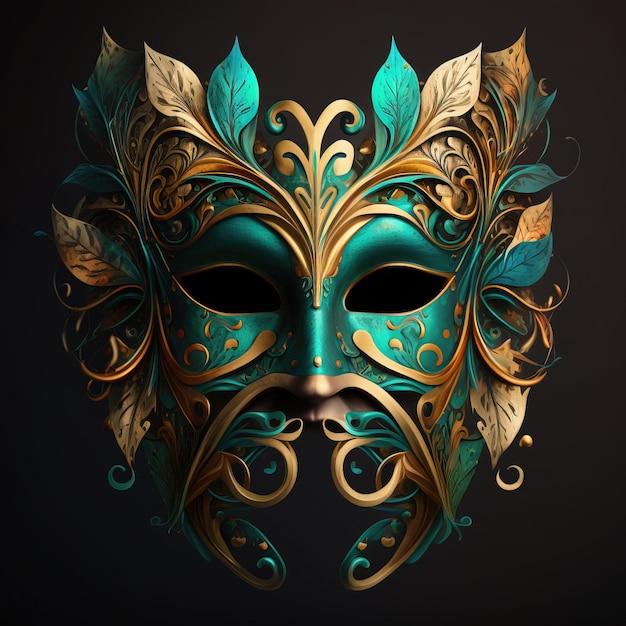The image depicts a decorative masquerade mask, predominantly teal blue with extensive gold embellishments. The mask is designed to cover just the eyes, which are cut out and appear as black shapes that tilt up to the sides. The metal-like mask features intricate scroll patterns and swirling designs in both teal and gold, particularly around the mouth and above the bridge of the nose. The edges and top of the mask are adorned with an array of teal and gold leaves, creating a fanned-out effect. The right side of the mask has a visible shine, while the left side is shaded. The entire composition is set against a dark gray background, enhancing the vividness of the mask's colors and details.